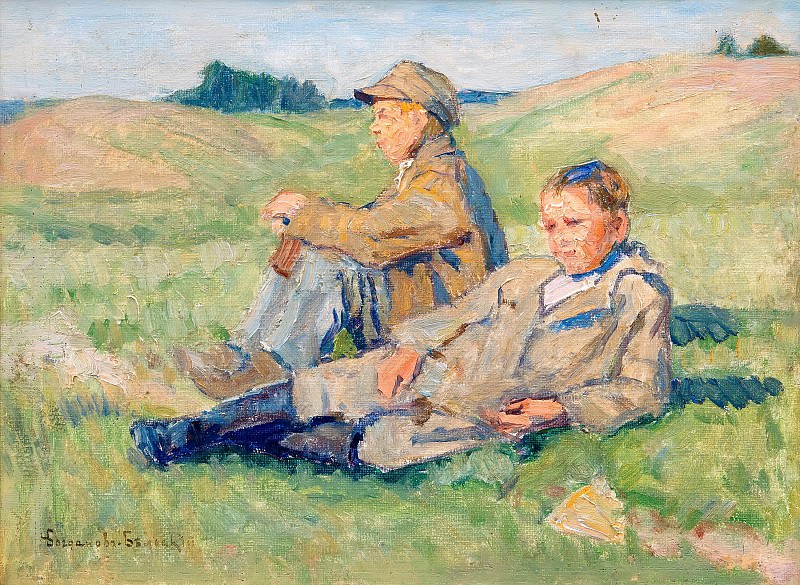The painting, rendered in an impressionist style, depicts a serene scene featuring a father and his preteen son in a rectangular frame. Both white-skinned with peachy undertones, they are positioned in the middle of the painting, set against a hilly background comprised of green and brown terrain with patches of a light blue sky and white clouds.

The father, seated and facing towards the left, wears a brown jacket, a matching hat, grayish pants, and brown boots. His hands rest on his knees in a relaxed manner. Beside him, the son stands on his right, capturing the viewer's attention with his contemplative gaze into the distance. He is dressed in a light brown coat with visible hands, blue pants, and tall black boots; he has short brown hair, with a peculiar blue spot atop his head.

The field they rest in is lush and green, dotted with the impressionistic brushstrokes that characterize the painting. In the background, subtle outlines of trees are visible against the rolling hills. The artist’s signature is inscribed in the lower left-hand corner, although it remains illegible.